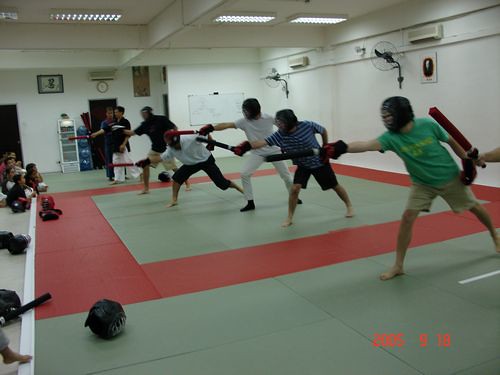The photo depicts a martial arts or self-defense class inside a gym with white walls and fluorescent ceiling lights. Central in the image are 6-7 individuals, each positioned on green and red mats that feature a red square outline. These participants, seemingly young people, are lined up next to each other, facing left with their right foot forward and left foot back. They are all captured in mid-action, lunging forward while gripping black batons or sticks in their right hands, with their left arms positioned at their sides. Each person is wearing black helmets with silver caged masks that cover their faces. Additionally, there are smaller children seated on the floor in front of them, attentively watching the demonstration. In the bottom-right corner of the photo, a timestamp reads "2005-9-10."